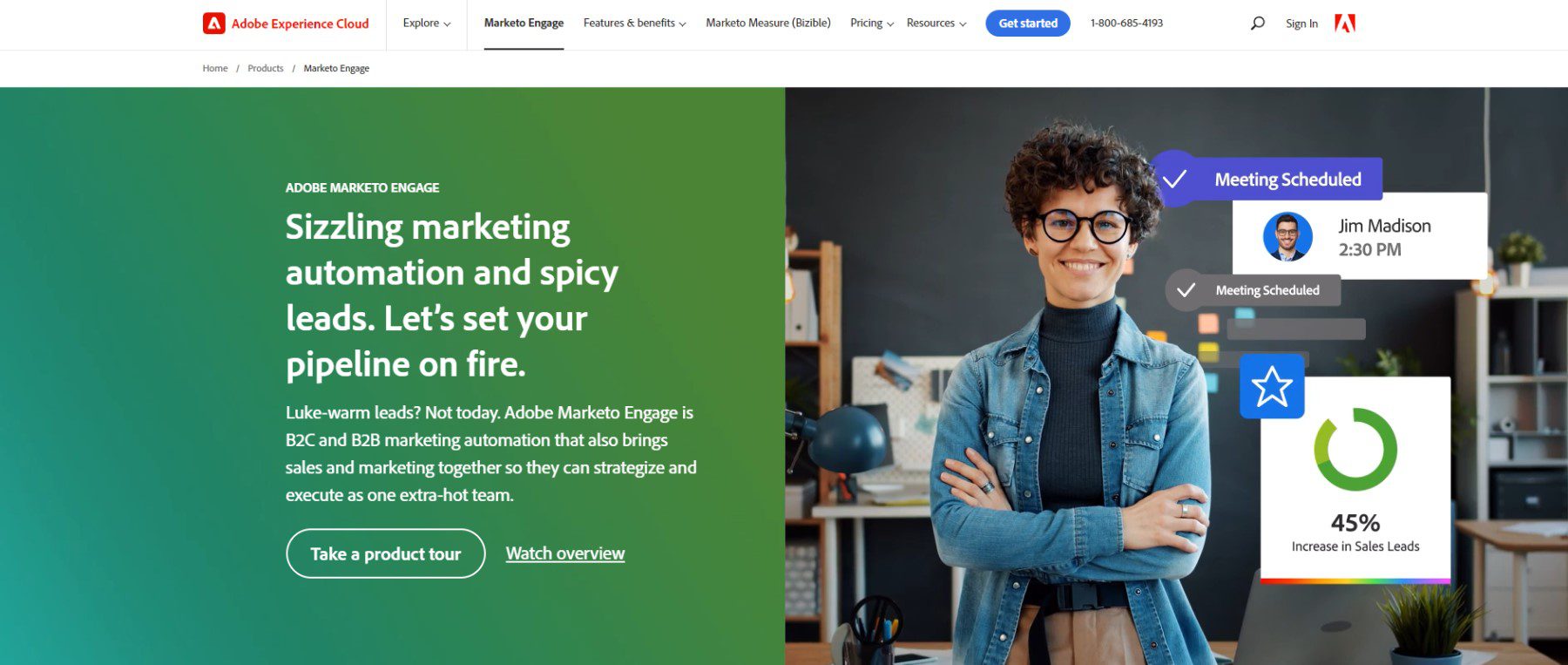"Screenshot of the Adobe Experience Cloud website, showcasing a welcoming banner image. On the right side of the banner, there is a young to middle-aged woman with short, curly hair, wearing brown-black glasses. She is smiling at the camera with her arms crossed. She is dressed in a blue turtleneck sweater under a denim jacket with blue pants. Next to her, graphics display messages such as 'Meeting scheduled with Jim Madison at 2:30 p.m.' and '45% increase in sales leads.'

On the left side of the banner, text reads: 'Adobe Marketo Engage. Sizzling marketing automation and spicy leads. Let's set your pipeline on fire.' Below this text, there is a button labeled 'Take the product tour' and a hyperlink on the right that says 'Watch overview.'

At the top of the webpage, a navigation bar includes tabs labeled: Explore, Marketo Engage, Features and Benefits, Marketo Measure, Bizible, Pricing, and Resources. There is also a blue 'Get Started' button, followed by a phone number, a search icon (magnifying glass), 'Sign In' text, and the red Adobe logo."